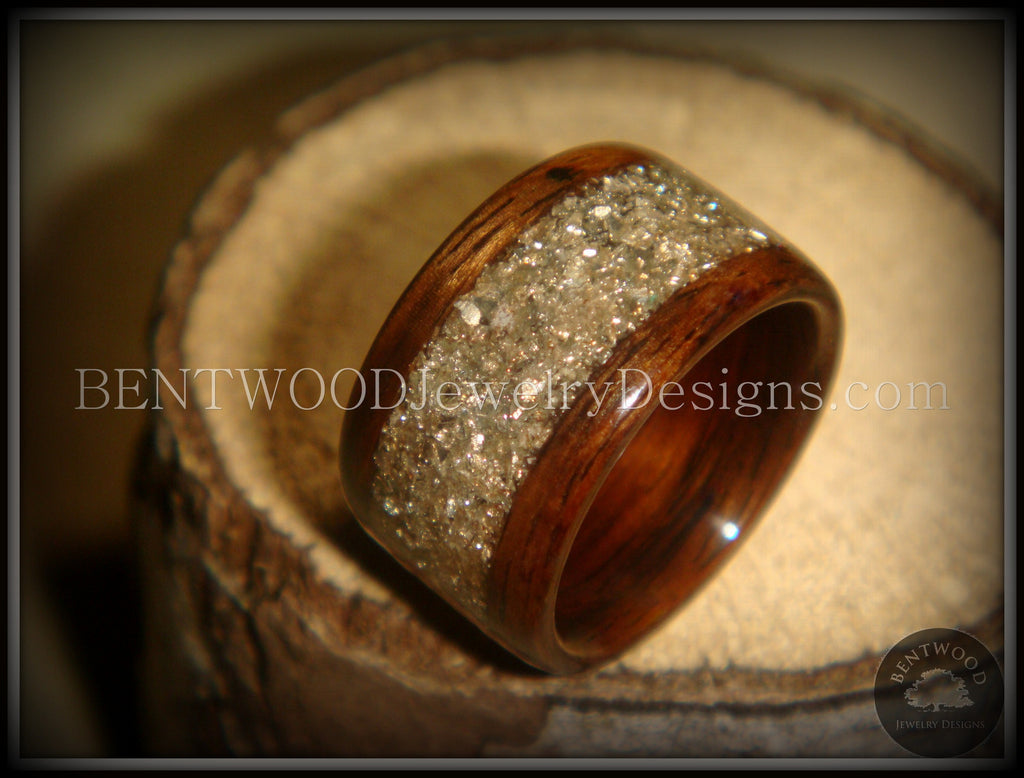The image features a detailed close-up of a wide band ring, meticulously crafted from rich brown wood with a discernible grain pattern. The wooden ring is adorned with a central line of white crystals or diamonds, artfully wrapped around the band’s middle section, adding a touch of sparkle. The ring sits elegantly on what appears to be a wooden or stone background, enhancing its rustic yet sophisticated appearance. The photograph captures the ring in bright, natural light, highlighting its intricate details and ensuring clear visibility. At the center of the image, there is an overlaid watermark that reads "bentwoodjewelrydesigns.com," and in the bottom right corner, the logo of Bentwood Jewelry Design is visible—a circle featuring a tree silhouette with the words “Bentwood” above and “Jewelry Designs” below it. The entire image includes a subtle black and gray border, framing the scene effectively.